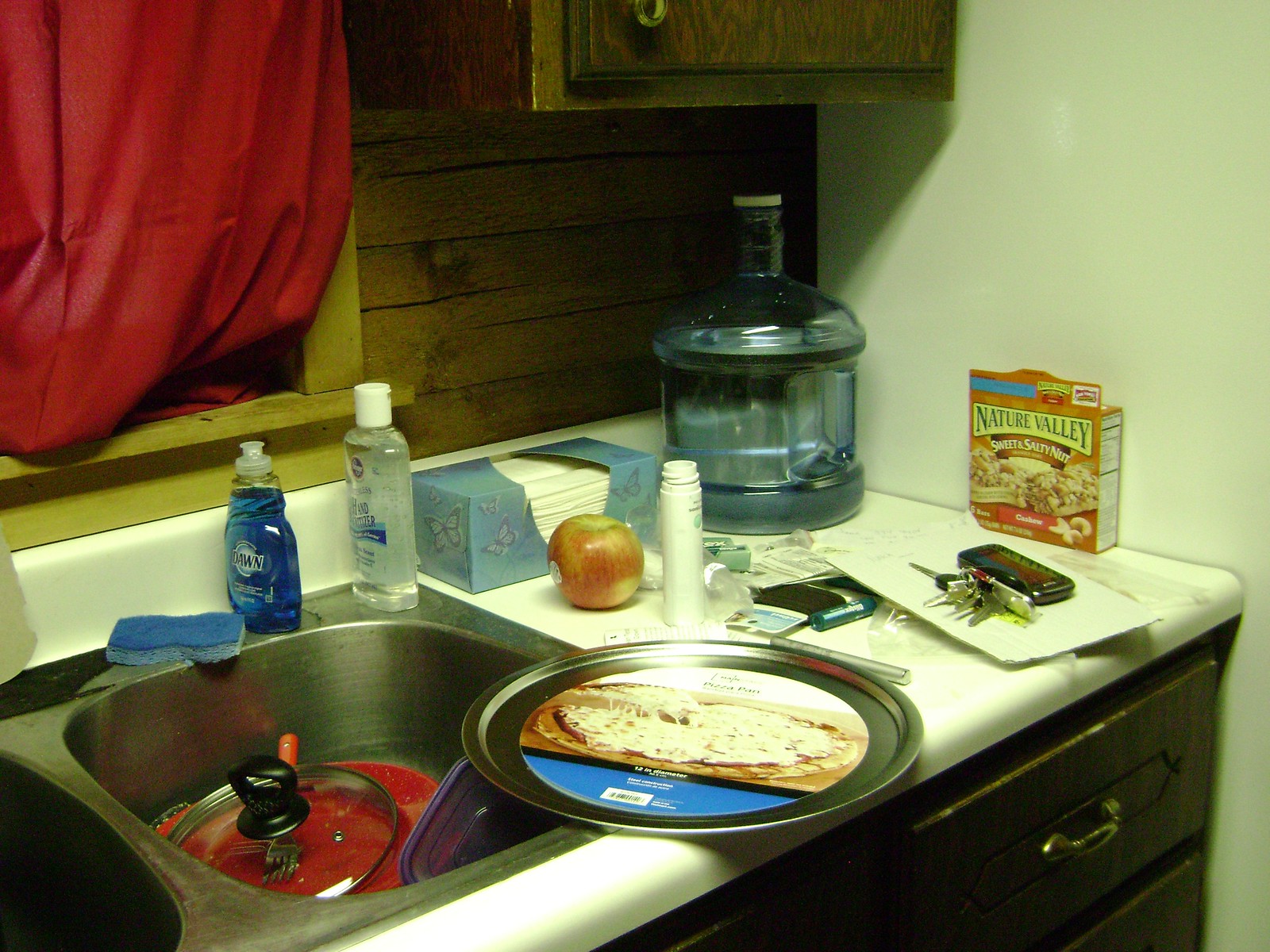The image captures a well-lived-in kitchen sink area, brimming with everyday essentials and details that tell a story. Centered in the background is a window adorned with a red drape, which appears to be casually tucked into the windowsill. The backdrop features a rustic backsplash comprised of old, splintered wood. Above this, the lower portion of a brown hanging cabinet is visible, accented with a silver handle in the bottom left corner.

On the countertop to the left, there is a very large, multi-gallon water bottle. This bottle, about three-fourths full, has a narrow top with a white cap and expands slightly wider towards the base. Positioned next to the water bottle is an open box of Nature Valley Sweet and Salty Bars, showing a hint of its nutritional information alongside the front of the box.

Further along the countertop, a cell phone rests on top of an envelope, accompanied by a set of keys nearby. A container of Blistex chapstick is also present, along with a white bottle standing upright. Behind these items, an apple with a sticker can be seen. The rear of the countertop features a long, narrow box of tissues, decorated with a light blue design and butterflies.

Below this array, the kitchen sink contains a bottle of hand sanitizer and a Blue Dawn soap dispenser. Inside the silver sink, a blue sponge lies alongside a pot lid, a red plate, and a Tupperware container. Balanced precariously between the counter and the sink is a pizza pan, still brandishing its original label.